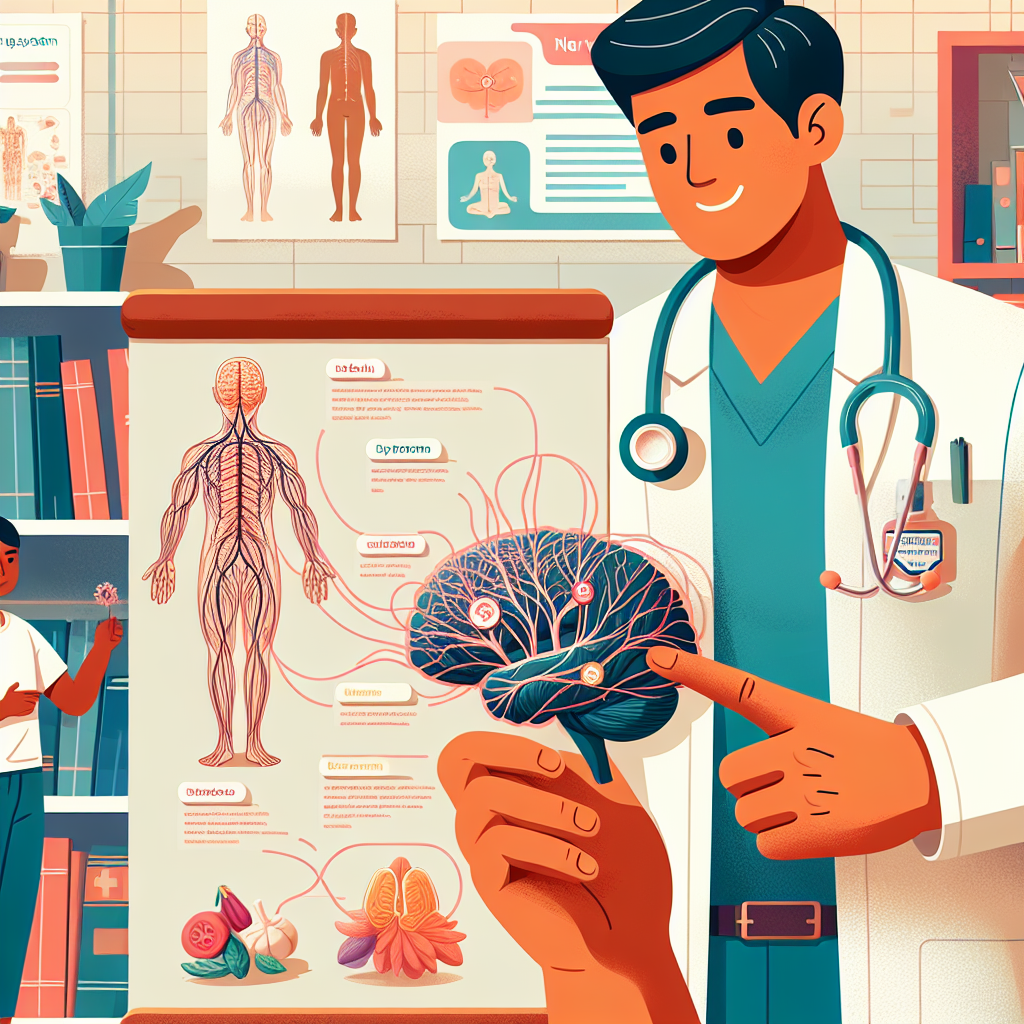This is a detailed digital illustration of a doctor in a clinical setting that resembles a doctor's office and library. The doctor, a man with short black hair and black eyebrows, stands on the right-hand side, wearing a traditional white lab coat over blue scrubs, a black belt, and a blue and red stethoscope around his neck. He is smiling and pointing at a detailed diagram of a blue brain with pink nerves, which is being held by an unseen hand.

In the background, there's a series of posters displaying scientific diagrams, including a human nervous system with labels and a diagram of fruits and vegetables at the bottom. Also visible are two bookshelves filled with books and some plants. The shelves are positioned on either side of the image, contributing to the scholarly ambiance of the scene. 

Additionally, there is a dark-skinned man partially visible on the left side of the image, holding a pink flower. This individual is wearing a white t-shirt and jeans, but parts of his body are cropped out by the edge of the image. Overall, the scene is rich with educational materials and anatomical illustrations, emphasizing the doctor’s role in explaining complex medical information.